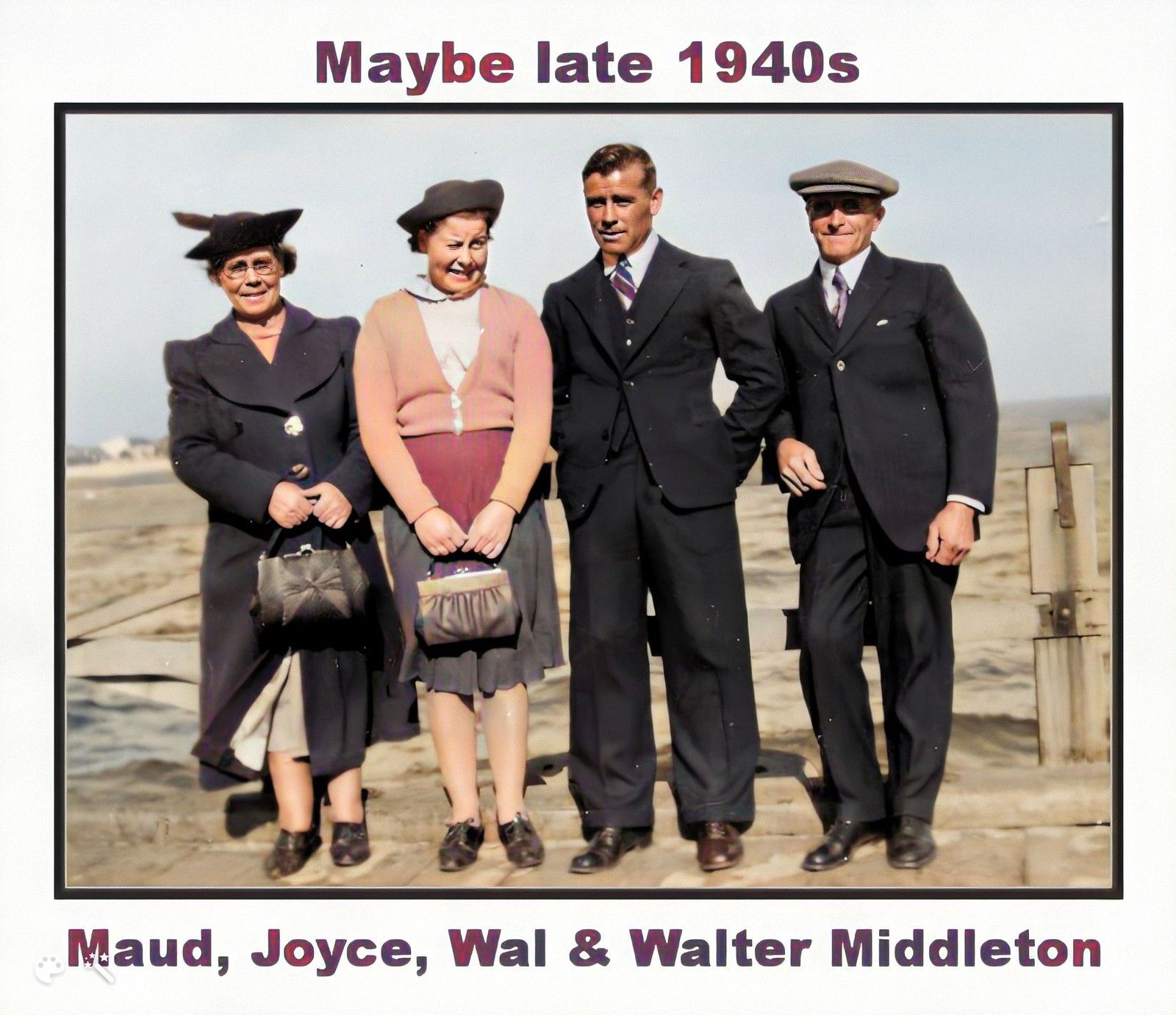This color photo, likely from the late 1940s, features four people posing outdoors in front of a barren, brown piece of land. At the top of the photo, the text reads "maybe late 1940s," while the bottom is labeled with the names "Maude, Joyce, Wall, and Walter Middleton."

From left to right:
- Maude is wearing a dark overcoat and a black hat, holding a taupe-colored purse in front of her. Beneath her coat, a khaki-colored skirt is visible, and she is wearing black shoes.
- Joyce stands beside her, dressed in a dark skirt that transitions from red at the top to gray near the bottom. She pairs this with a coral pink cardigan over a light-colored shirt, and she also wears a dark gray hat and taupe-colored purse, with black shoes completing her outfit.
- Next to Joyce stands Wall, dressed in a three-piece dark suit with brown shoes. He sports a blue and purple striped tie.
- Finally, Walter, also in a dark suit, is wearing a white shirt, a purple tie, black shoes, and a tan-colored hat.

The photo is surrounded by a white border.